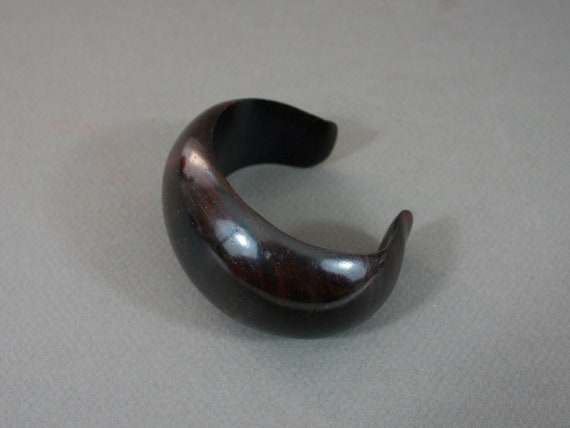The image features a deep brown wooden bracelet with a nearly black appearance, revealing intricate wood grain patterns and swirls upon close inspection. The bracelet captures reflections from photography lights, notably those within white umbrellas, indicating a professional shoot. It lacks ornamentation and suggests a vintage quality with visible signs of wear. Positioned at the center of the image against a gray fabric backdrop, the bracelet stands out with its translucent sheen where light hits it in three distinct spots. The bracelet appears slightly open, revealing a gap that suggests a loose fit. The overall muted tones of deep brown and gray emphasize the bracelet's details and craftsmanship, making it the focal point of what seems to be a professionally styled product photograph.